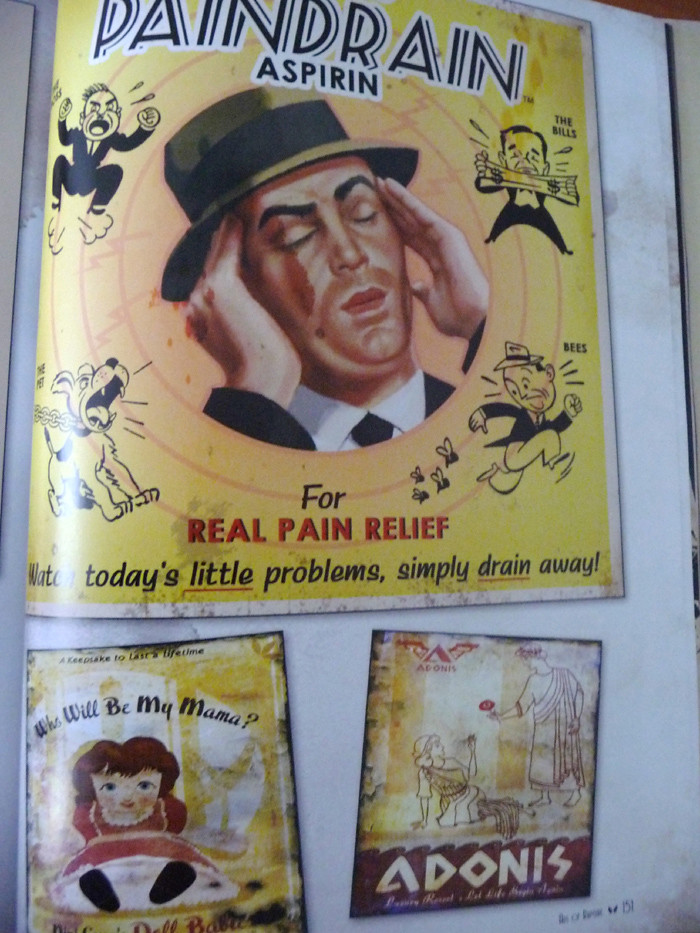The image depicts a vintage magazine advertisement for Pain Drain Aspirin, prominently featuring a Caucasian man wearing a fedora and a suit with a tie, holding both hands to his brow, ostensibly to indicate a headache. The top of the ad reads "Pain Drain Aspirin" in black text against a yellow background, accompanied by cartoon depictions of various stressful scenarios, including a man jumping in anger, financial distress, and a person fleeing from bees. Below the man's image, the ad promises "For real pain relief" in red text and states, "Today's little problems simply drain away!"

The bottom section of the ad includes two additional advertising images. On the left, an ad for a doll features a young girl with the caption "Who will be my mama?" On the right, a drawing of two individuals in togas—one of whom is labeled "Adonis"—is seen. This detailed layout provides a glimpse into historical advertising methods and the everyday concerns they aimed to address.